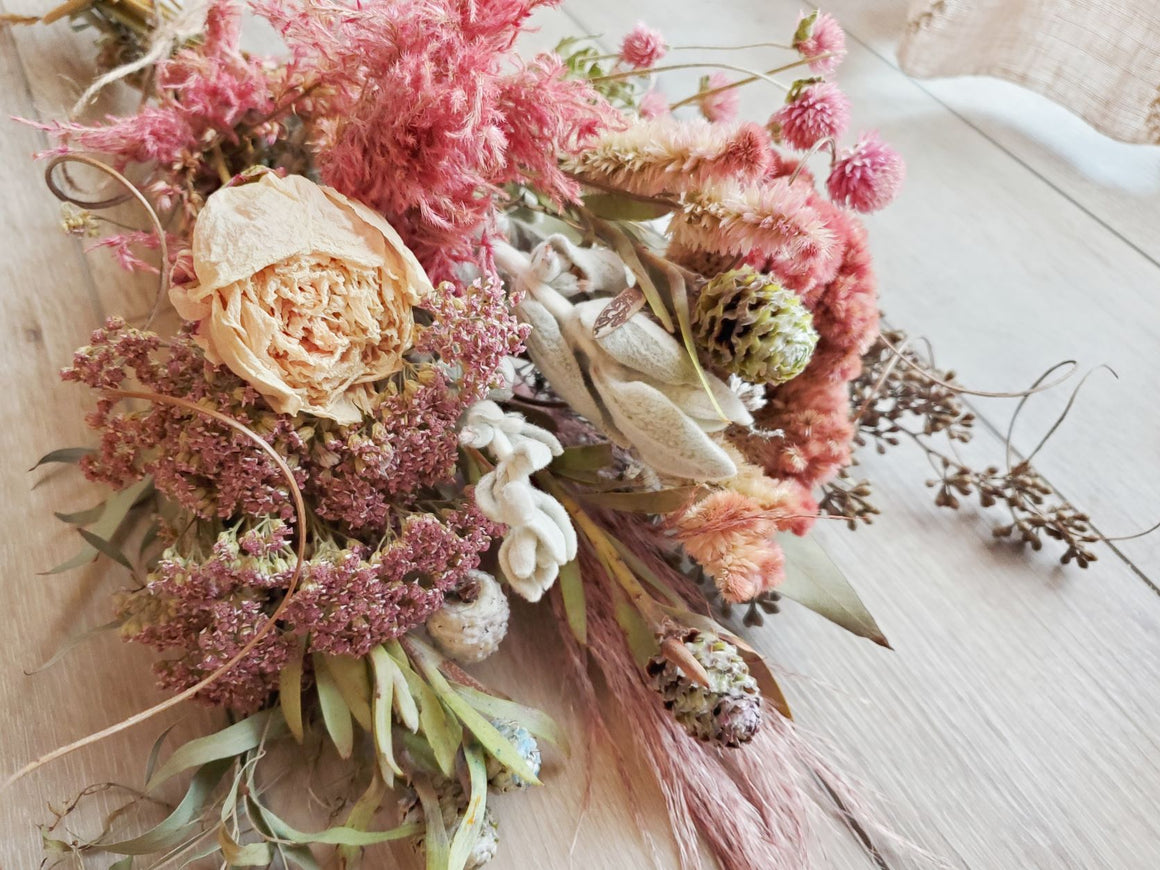This detailed photograph depicts a vibrant and meticulously arranged bouquet of dried flowers resting on a white wooden table, evoking a beachy, sunlit vibe. The elongated, vertically-run planks of the table lend a sense of depth to the scene. The bouquet, which occupies the majority of the image, combines a mix of colors and textures: prominent, fluffy pink flowers reminiscent of pampas grass, delicate purple blooms, a light pink or white rose, and several smaller white flowers with elongated petals. Adding to the variety are some earthy brown elements and a few green leafy sprigs that stand out at the base. The arrangement is further enhanced by the presence of pinecone-like objects and twiggy branches. In the background, to the left, a hint of a linen curtain bathed in sunlight adds a serene, homey touch, making the scene reminiscent of springtime or a romantic wedding.